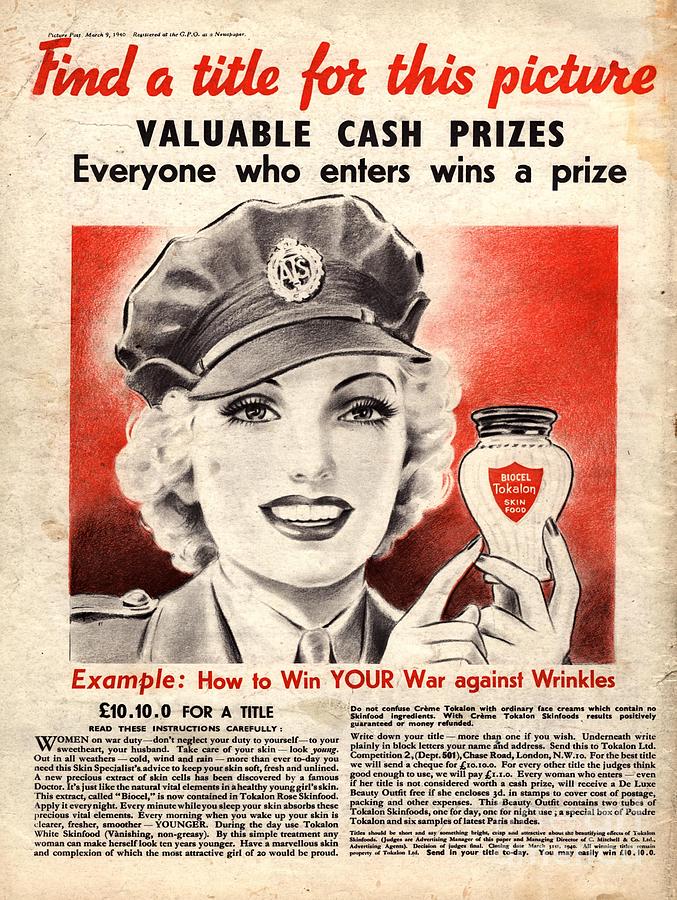This vintage advertisement, likely a page from a magazine, features a war-themed recruitment poster repurposed for a skincare product. The poster has a light brown background and prominently displays a blonde woman with curly hair, adorned in a pilot's hat with a gold emblem, and dressed in a soldier's uniform with a collared shirt and tie. She is smiling and holding a bottle labeled "Biocell Tecalon Skin Food." At the top, in bold red text, it reads, "Find a title for this picture," followed by the promise of "valuable cash prizes" in black text, with the note that "everyone who enters wins a prize." Beneath the woman, the slogan declares, "How to win your war against wrinkles," enticing readers to participate in a contest for a prize of 10 pounds. The ad hints at additional instructions in fine print that are not entirely legible.